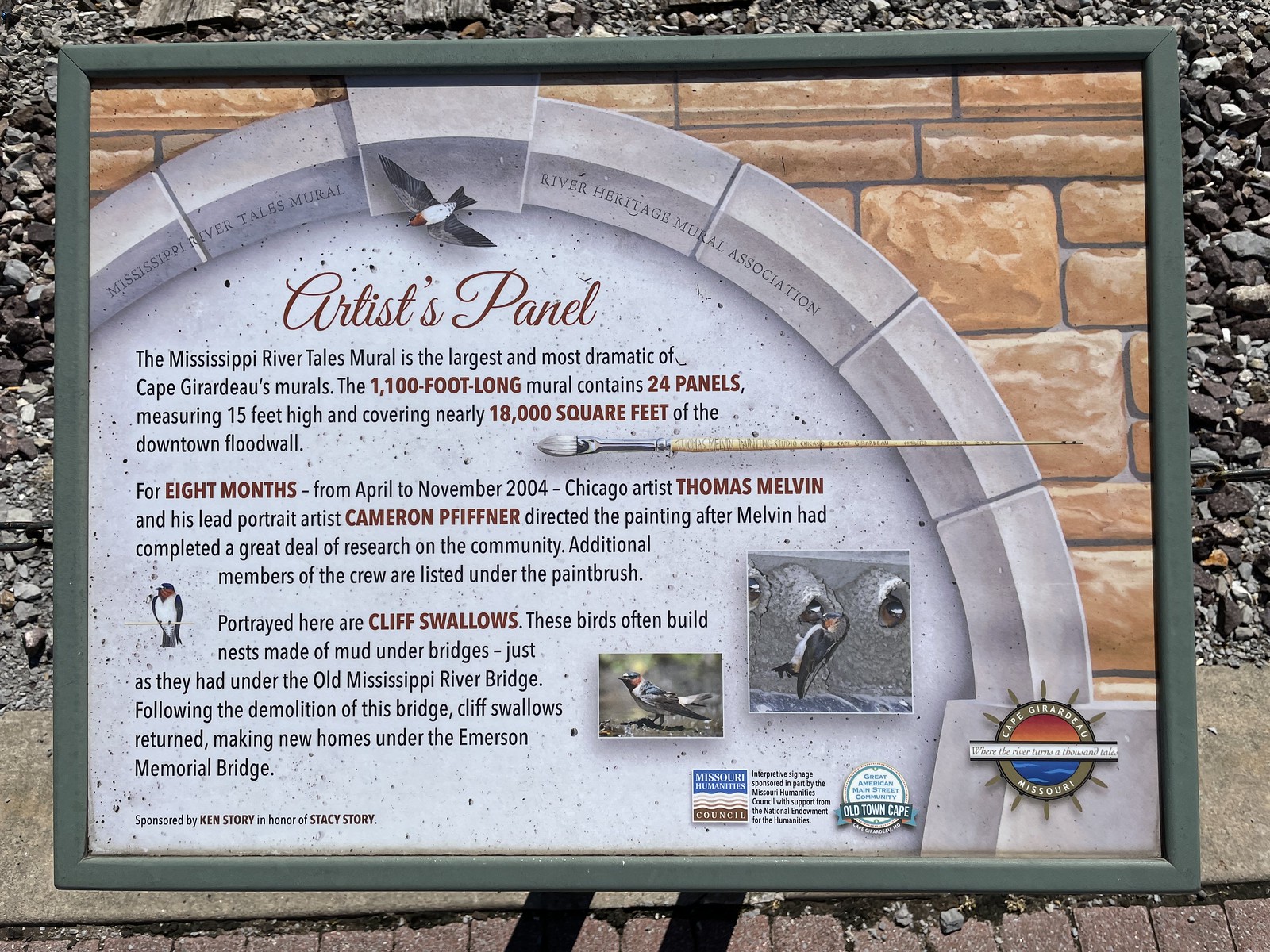This photo captures an information plaque set against an outdoor backdrop, featuring a gravel-like path and a sidewalk at the bottom. The plaque, titled "Artists Panel," provides detailed context about the Mississippi River Tales Mural, hailed as the largest and most dramatic of Cape Girardeau's murals. Spanning 1,100 feet and composed of 24 panels each measuring 15 feet high, the mural covers nearly 18,000 square feet of the downtown flood wall. The creation process, directed by Chicago artist Thomas Melvin and his lead portrait artist Cameron Pfeiffer, spanned eight months from April to November 2004, following extensive community research by Melvin. Additional crew members are acknowledged under a paintbrush motif on the plaque. The plaque also features an image of cliff swallows, illustrating a narrative about these birds building nests under the old Mississippi Bridge and later the Emerson Memorial Bridge. Various logos, though not fully legible, are visible at the bottom of the sign. The setting is accentuated by the presence of the sun in the background and a wall composed of compressed rocks.